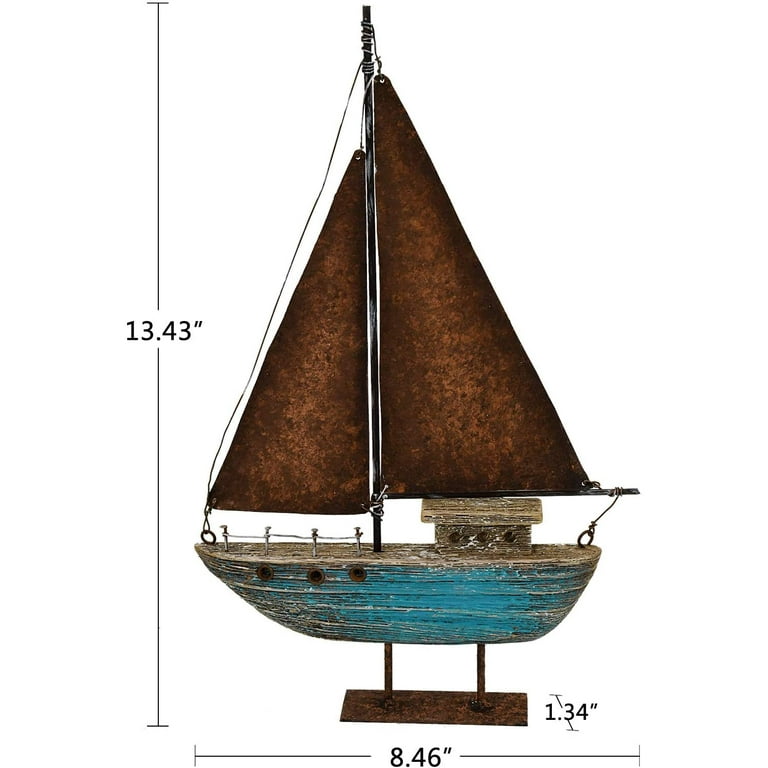This detailed photograph showcases a meticulously crafted wooden model sailboat perched on a metal stand. The base is made of copper, featuring two poles that support the boat. The hull is carved from a block of wood and painted blue, with the paint visibly fading at the edges. The boat measures 13.43 inches in height, 8.46 inches in length, and 1.34 inches in width, as indicated by thin lines with numerical annotations on the image. A small miniature cabin is situated on the right side of the hull. The model's sails are a dark brown, resembling parchment, and are held up by a metal mast. The backdrop of the image is a plain white, with no border, emphasizing the boat's intricate details and craftsmanship.